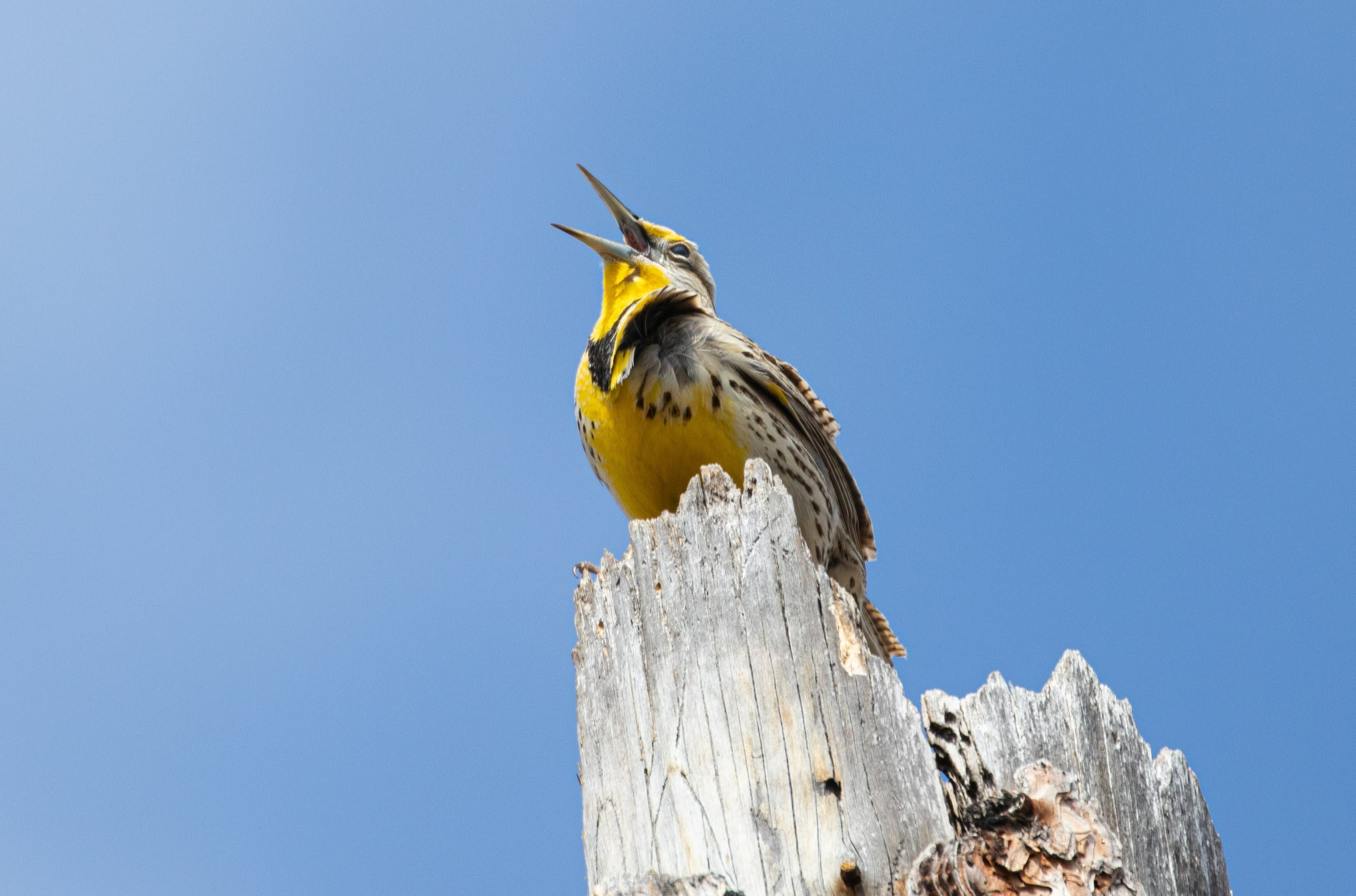Captured in brilliant daylight under a clear blue sky, this high-definition wildlife photograph showcases a striking scene of nature. The background features a bright blue sky that is slightly more saturated on the right side, hinting at the sun's position to the left. At the bottom right corner of the rectangular frame, a weathered, jagged tree trunk emerges, about two inches wide at the base, its grayish, rotted surface conveying the passage of time.

Resting majestically atop the tree trunk is a large yellow bird, its vibrant colors illuminated by the sunlight. The bird faces left, its head tilted back and mouth open, revealing its long, pointed beak that is white with black tips. Its crown, throat, and belly are a vivid yellow, contrasting starkly with the black 'scarf' of feathers around its neck. A gray stripe adorns the area between its eye and throat, adding to its striking appearance. The bird's underside is dotted with black spots, while the sides feature white feathers with black and brown specks. Its tail, visible from the viewer’s vantage point looking up, is composed of long white and brown feathers. The photograph captures the essence of this bird in its natural habitat, frozen in a moment of expressive vitality.